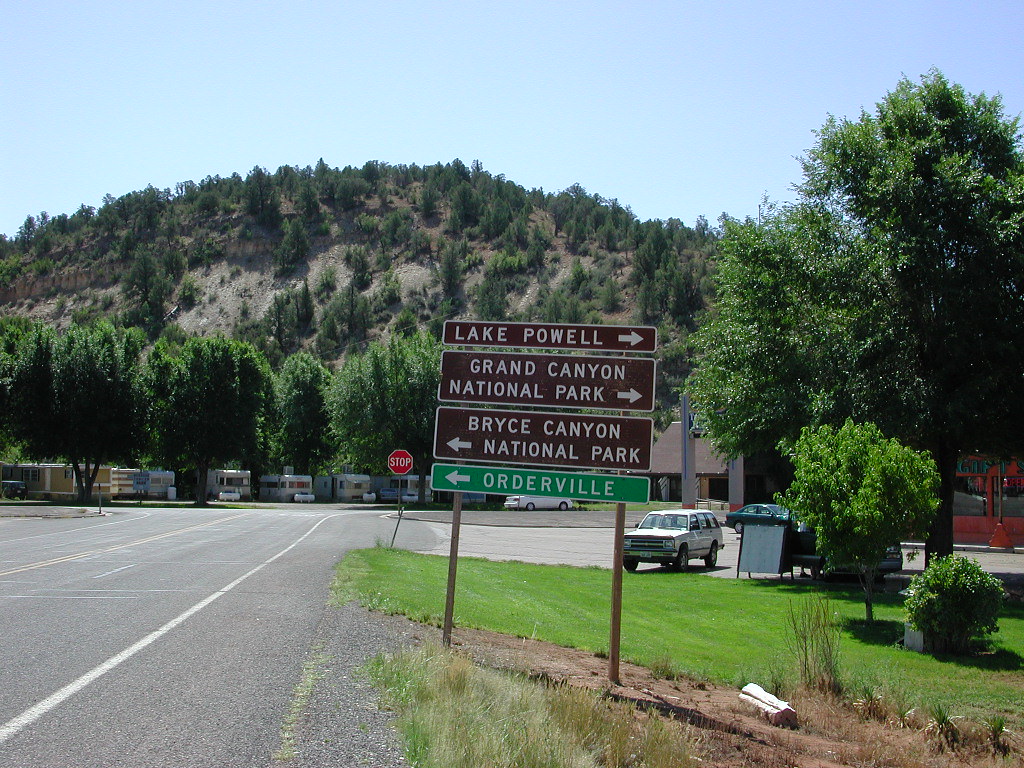This detailed photograph captures a road sign situated against the backdrop of a mountain landscape on a clear day. The signpost, standing on two wooden legs, displays four directional signs. The topmost brown sign with white text points to the right and reads "Lake Powell." Below it, another brown sign directs to the right towards "Grand Canyon National Park." The third sign, also brown, indicates a left turn for "Bryce Canyon National Park." The bottom-most green sign with white text points left to "Orderville." Around the signpost, there is a road veering left with a few cars, some old-school SUVs, motorhomes, and a stop sign visible. The scene includes elements of greenery with trees, grass, and some scattered garbage on the asphalt. The entire scene is framed by towering mountains in the background and is set under a blue sky dotted with white clouds, giving a sense of a serene and open landscape.